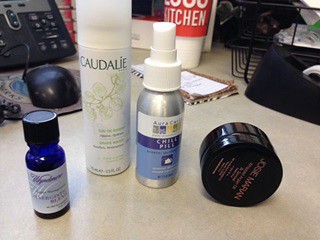The image features a variety of items arranged in a specific order. Starting from the left, there is a small, dark blue bottle with a black lid. The bottle has cursive text in purple, which is very small and hard to read, against a white background. To its right, there stands a tall, white aerosol-like can with the word "CAUDALIE" prominently displayed, along with an image of a plant. While there is additional text beneath, it is illegible in the image. Next, we see a small sterling silver spray bottle, characterized by its white spray nozzle at the top. Finally, there is a black jar, approximately three inches in length, lying on its side. The jar's lid features some pink text.

In the background, towards the far left corner, there appears to be a telephone or answering machine. Adjacent to this is a black computer mouse resting on a mouse pad. Further to the right, there is a tube labeled as a type of cleaner with the word "kitchen" visible at the bottom, and directly underneath this tube is a small white notepad.